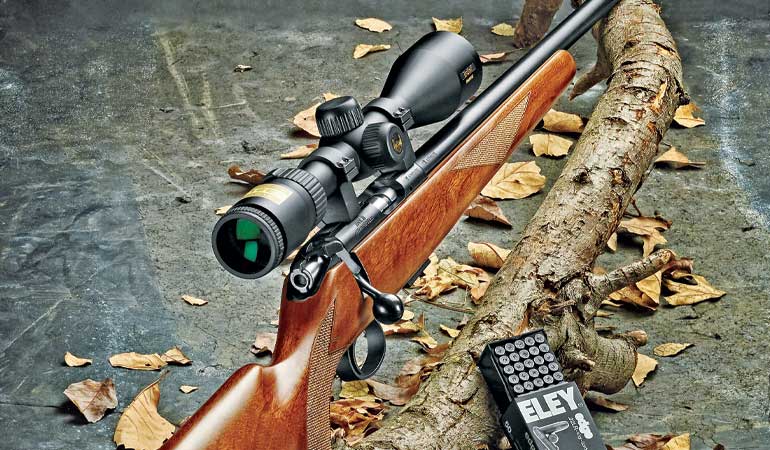This is an outdoor daytime photograph of a bolt action hunting rifle with a mounted scope, resting at an angle on the ground against a small tree branch. The rifle features a brown stock and a long barrel, with a visible lever on the side, confirming its bolt action mechanism. Positioned next to the rifle is a partially open black box of ELEY brand bullets with white writing, resting against the tree branch to display the cartridges inside. The scene appears to take place on hard-packed dirt, surrounded by natural elements. Unexpectedly, inside the scope where one might look through, there are what appear to be apple slices, an unusual detail that stands out in the image. The colors present in the photo include various shades of brown, black, green, white, and gray.